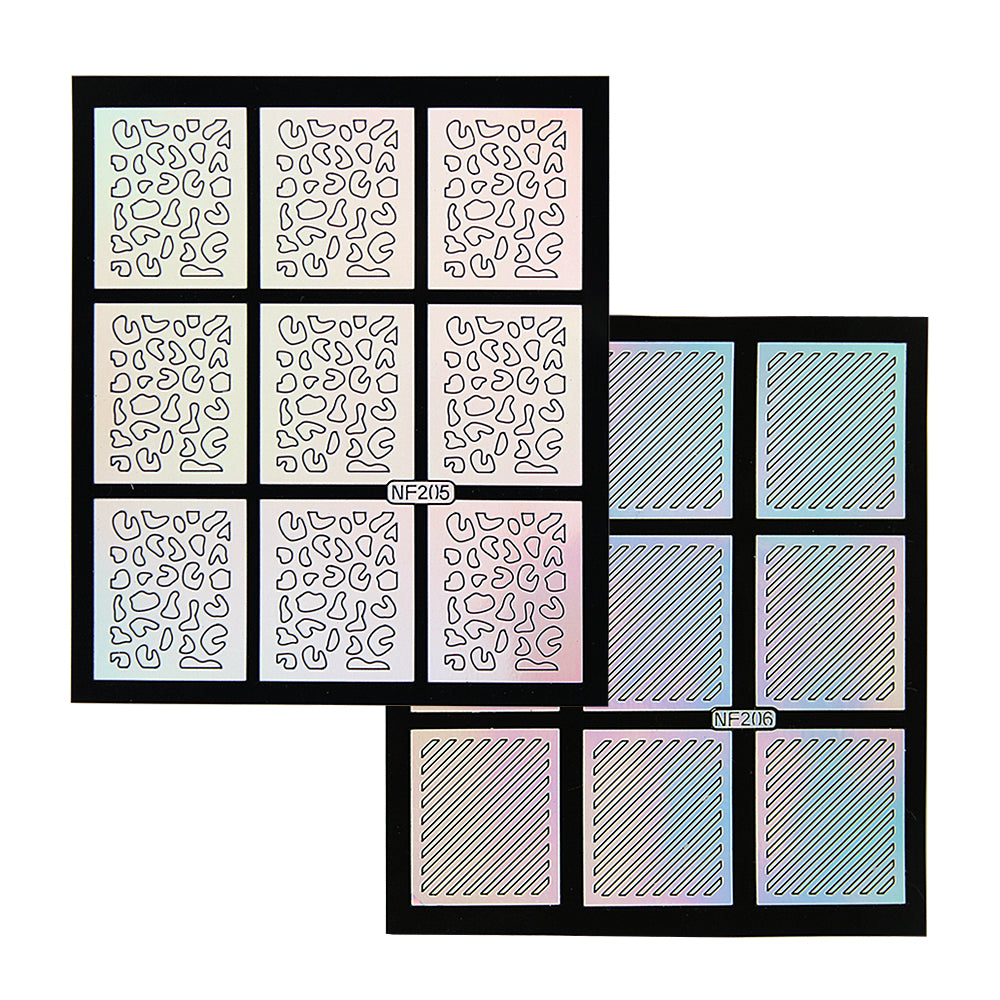The image features two distinct sections, each composed of a 3x3 grid of smaller images, totaling 18 individual images. The top left section is labeled NF-205 and contains designs with an underlying pattern of black frames. Inside each of these frames, various abstract shapes and squiggles, somewhat chaotic and random in appearance, fill the spaces. This section tends to have a grayscale color scheme with some light pinkish tones and patterns resembling leopard designs. Off to the right, in the section labeled NF-206, the grid follows a similar 3x3 arrangement. These images are more meticulously organized with diagonal lines set against light bluish backgrounds. Both sets maintain the same structural layout but differ significantly in color scheme and design intricacy, with the right set appearing more orderly and deliberate in its execution.